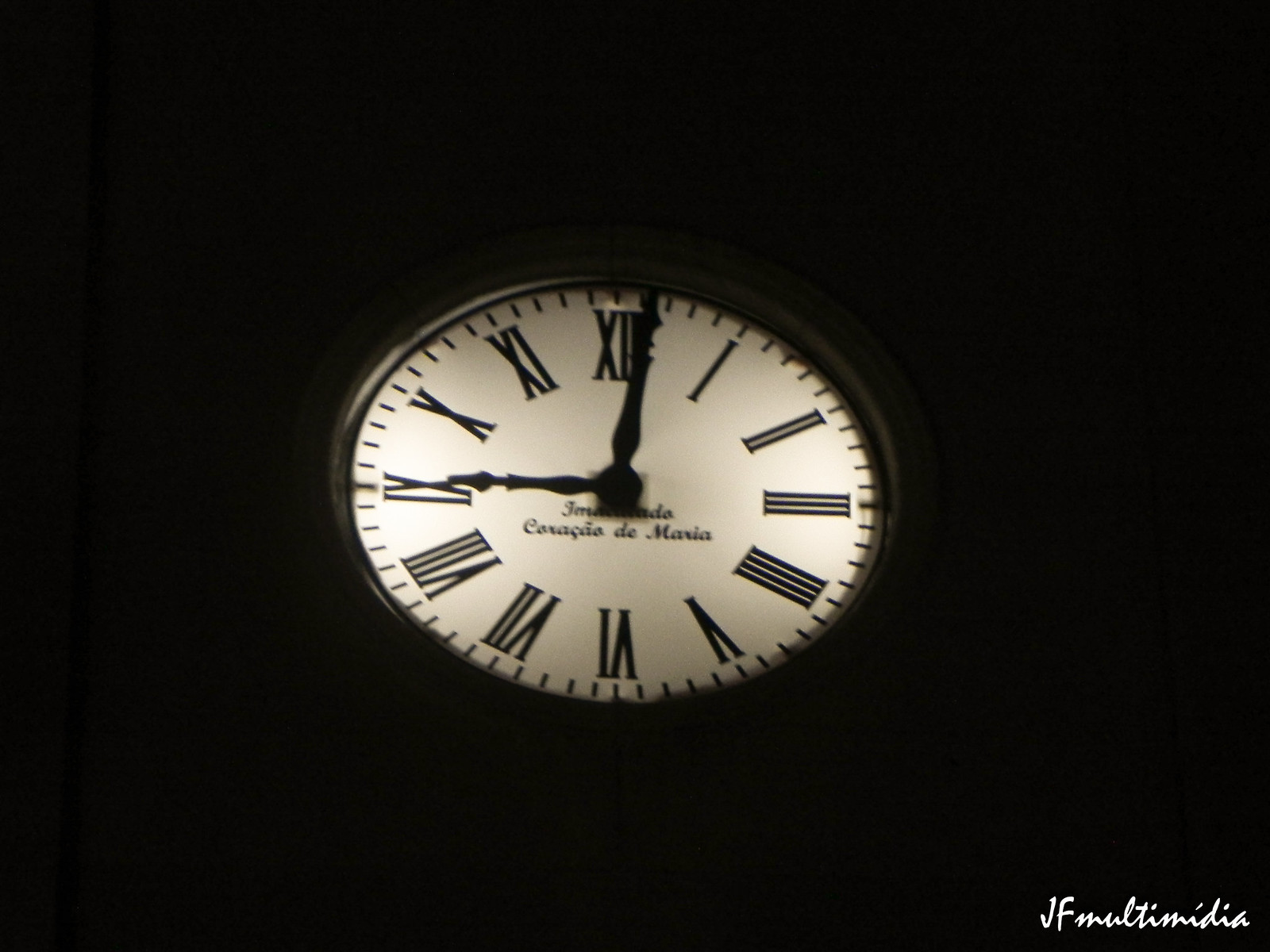This is an outdoor nighttime photograph featuring a large round clock face, likely mounted on a building or pole, captured from a low angle that tilts the top slightly back. The clock displays a time of 9:01 and has a white face illuminated from behind. The clock's numerals are black Roman numerals, and the minute markers are black dashes. The clock hands are also black, and there is a cursive inscription under the hands, partially obscured by shadow. It reads "C-O-R-A-C-A-I-O-D-E-M-A-R-I-A". The entire background surrounding the clock is pitch black. In the lower right corner of the image, there's a white cursive text overlay that says "JF Multimedia". The clock face appears slightly blurred, adding a subtle soft focus effect to the photograph.